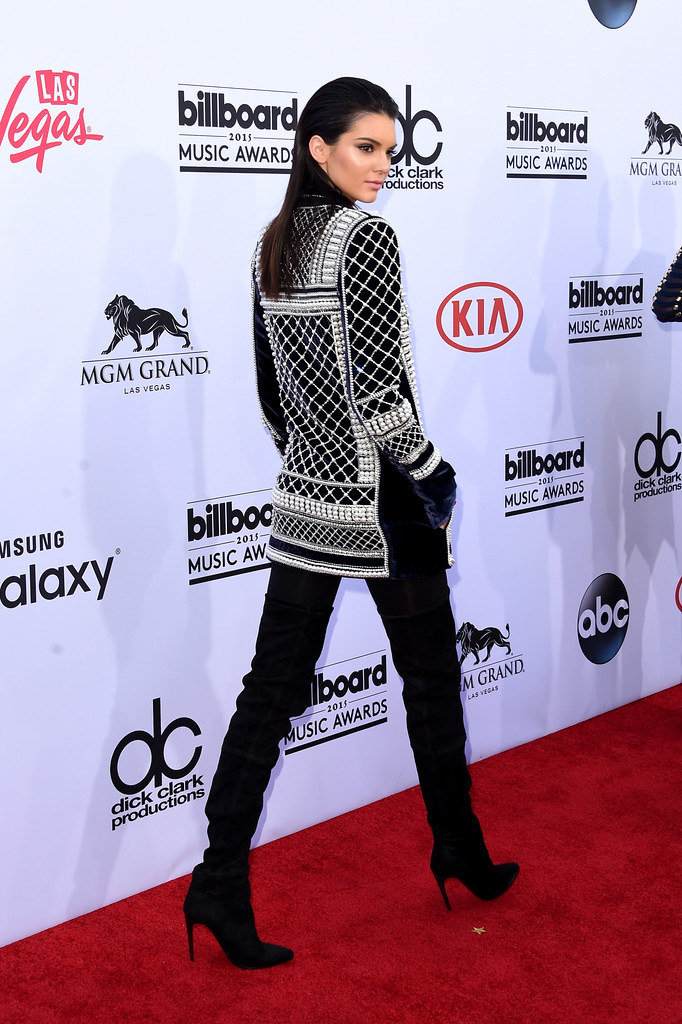Kylie Jenner is featured in a striking photograph taken at the Billboard Music Awards held at the MGM Grand in Las Vegas. Dressed in an eye-catching ensemble, she dons black high heels, black pants, and a stylish black and white checkered top. Her slicked-back hair accentuates her intense gaze towards the camera. She stands confidently on the red carpet, framed by a white backdrop adorned with numerous logos including the Billboard Music Awards, MGM Grand, ABC, Kia, Descartes Productions, Dick Clark Productions, and Samsung Galaxy. The vibrant red “Las Vegas” text adds a pop of color to an otherwise monochromatic scene, capturing the essence of the glamorous event.